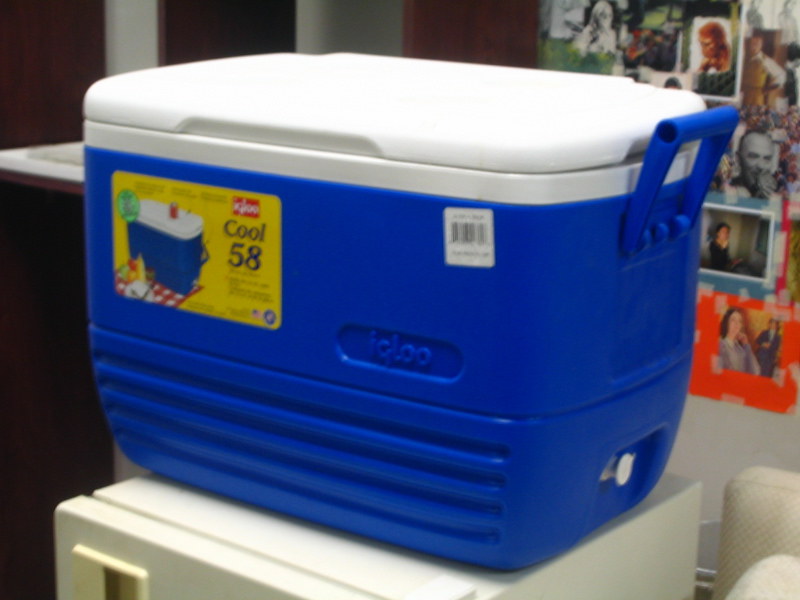This slightly blurry photograph captures a blue Igloo cooler prominently placed inside an interior room. The cooler features a white hinged lid, blue handles, and a white drain spout on its right-hand side. On the left side of the cooler, a yellow product sticker with a drawing of the cooler and "Igloo Cool 58" in black lettering is visible, while a price sticker and barcode are on the right side. The cooler is positioned atop a white dormitory-sized mini-fridge, which has a door hinged on the right. In the background, a collage of family photos is displayed on a white wall, and the lower right-hand corner of the photo shows a portion of a white armchair.